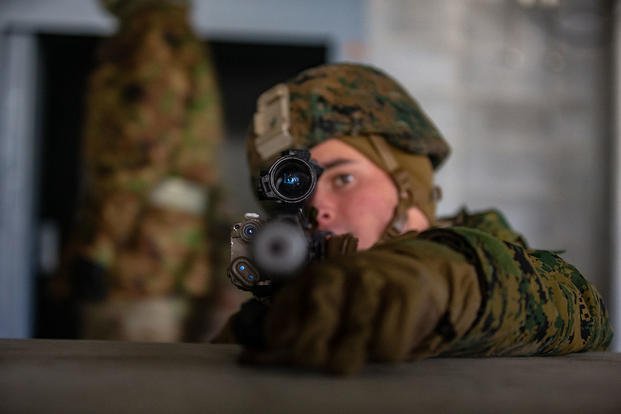This photograph captures a young soldier, around 20 years old, in full military gear, pointing his advanced sniper rifle directly at the camera. The image is taken from the perspective of looking down the barrel of the rifle, emphasizing the view through the telescopic scope. The soldier is dressed in a camouflage uniform, complete with a camouflage helmet that features attachments, possibly a light or sensor, and a chin strap. He is also wearing dark gloves and a greenish beanie underneath his helmet. The rifle appears complex, with visible features such as the scope and other advanced functionalities. He is resting his arm on a platform for stabilization. In the background, slightly blurred, another soldier in a camouflage uniform is seen, partly cut off from the neck down to the thigh, walking past a blurry white and grayish wall and doorway towards the left-hand side. This creates a dynamic and detailed military scene centered around the focus of the poised sniper.